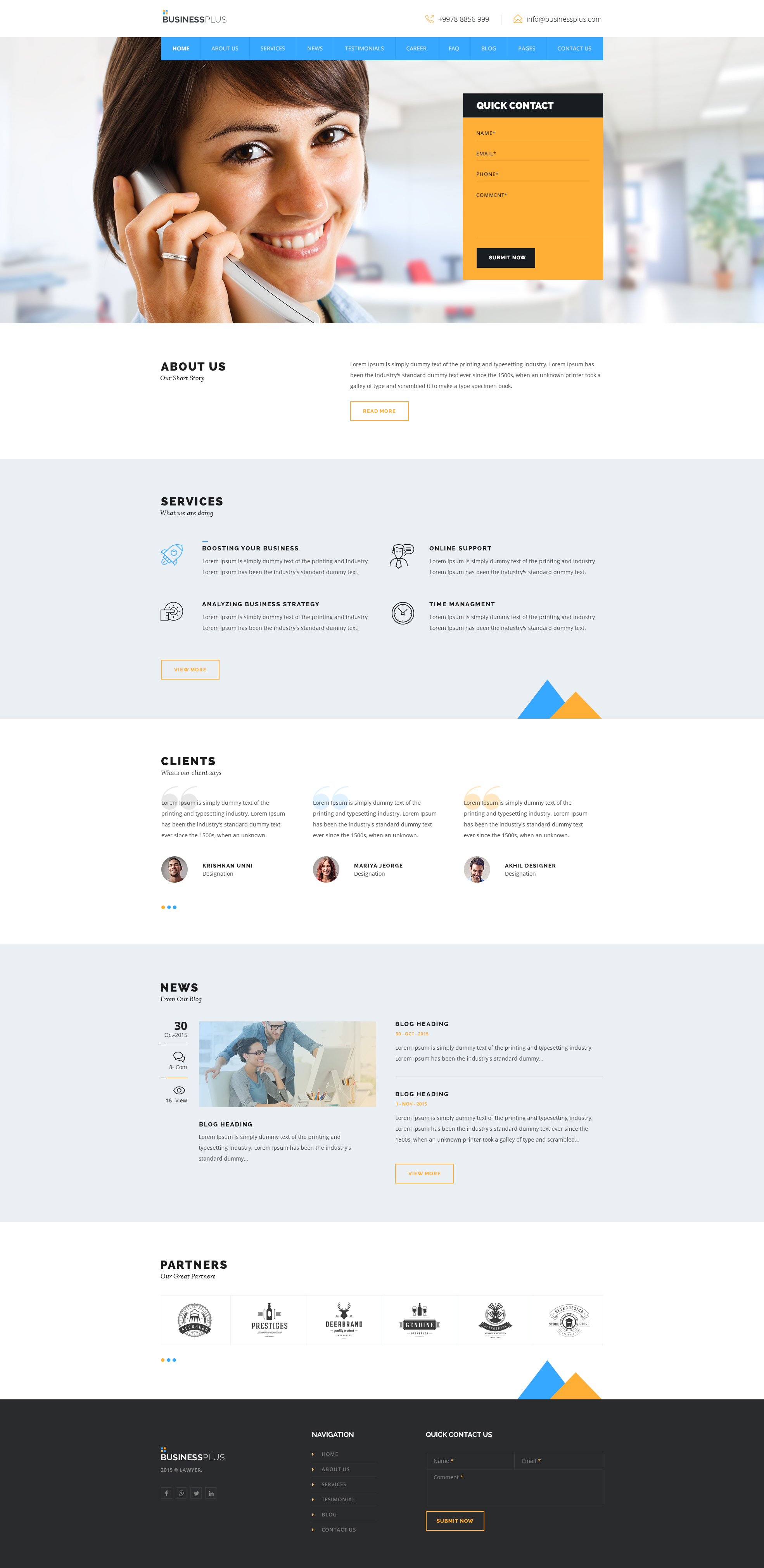The vertical screenshot features a website with various sections, although the exact URL at the top is too small to read. The page begins with a blue horizontal menu bar at the very top center. Just beneath this bar, there's an image of a woman smiling while holding a phone to her ear; she has short brown hair and her face is prominently displayed against a minimal background.

Adjacent to this image, a text box reads "Office Contact" followed by additional, smaller, hard-to-read text. Below this header, the section titled "About Us" appears, immediately followed on the right by some kind of explanatory text.

Further down, there is a "Services" section featuring four distinct services, each accompanied by a small icon. Following this, the "Clients" section is showcased, which includes three testimonials, each paired with a profile picture of the respective individuals. 

The subsequent "News" section contains an image of two people with several text boxes scattered around it. Lastly, at the very bottom of the webpage is a "Partners" section displaying a series of six logos. The page concludes with a black footer box.